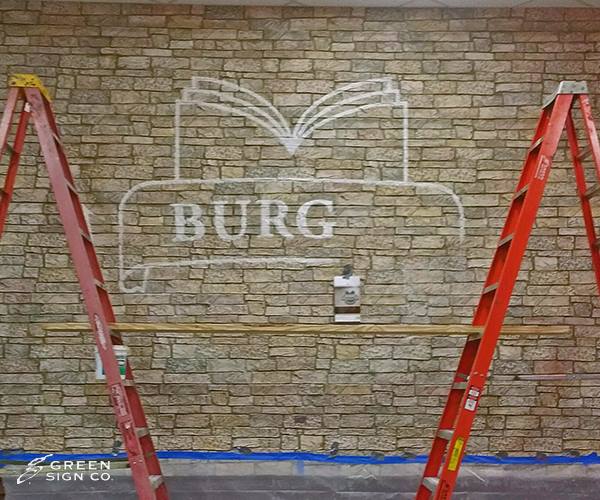The photograph shows a detailed indoor scene with artificial lighting, featuring a rugged stone wall composed of various horizontal, irregularly shaped rectangular stones. Centrally positioned on the wall is an unfinished painting. The upper part of this painting depicts the front view of an open book, executed in white. Below the book is a rectangular banner also outlined in white, bearing the partially painted word "B-U-R-G."

Flanking either side of the wall are two red step ladders, arranged in an inverted V-shape. A brown wooden board spans between the ladders, likely serving as a makeshift scaffolding for the painter, with a can of paint resting on it. 

At the lower left-hand corner of the image, toward the stone floor, a small piece of text added digitally reads “Green Sign Company,” with the "G" in a fancy lowercase cursive and the rest in all capital letters. The floor itself appears to be stone and includes a blue tape running vertically, separating it from the wall. Sprinkled with tones of gray, tan, brown, red, and white, the scene is vibrant yet industrial, providing a glimpse into the workspace and ongoing creative process of the painter.